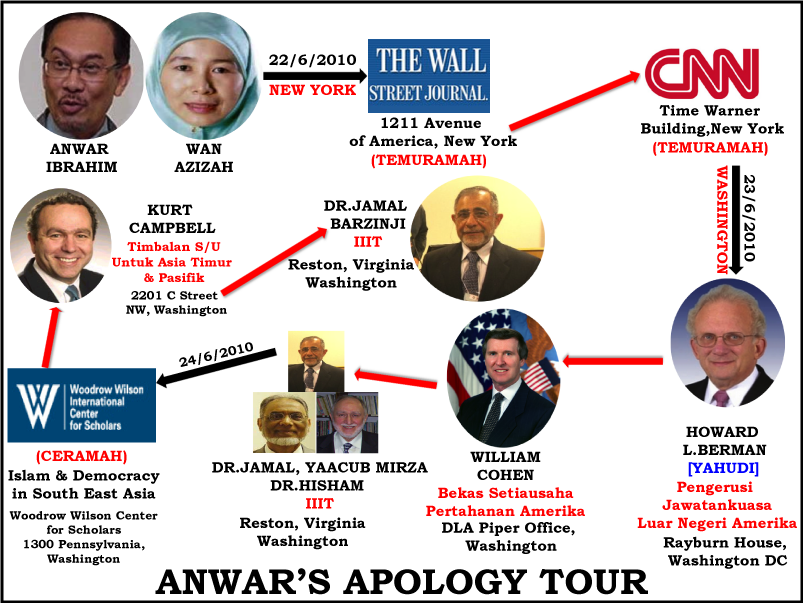The image is a detailed graphical representation titled "Anwar's Apology Tour," prominently displayed in black letters on a white background at the bottom center. The horizontal layout is slightly rectangular and features a series of interconnected round and square photographs, logos, lines, and text, forming a busy diagram.

In the upper left corner, there is a round photo of Anwar Ibrahim, an Asian middle-aged man wearing glasses, identified by his name beneath the photo. Adjacent to his photo is an image of Juan Aziza, an Eastern woman adorned with a headscarf, her facial features clearly visible, with her name also labeled below.

Starting from Anwar Ibrahim's photo, arrows guide the viewer through his itinerary. The first destination, marked by a date of June 22, 2010, is The Wall Street Journal office at 1211 Avenue of America, New York. Following the arrows to the right, the next stop is the CNN headquarters in the Time Warner Building, New York, indicated by the same date.

Continuing across the diagram, on June 23, 2010, in Washington, D.C., the itinerary reaches Howard L. Berman at the Rayburn House, followed by William Cohen, and then Dr. Jamal Yacoub Mirza and Dr. Hisham in Reston, Virginia. Each individual is portrayed with a portrait photograph alongside their respective names, titles, and locations. 

The tour proceeds to the Woodrow Wilson International Center for Scholars on June 24, 2010, specifically addressing Islam and democracy in Southeast Asia. The final stop involves Kurt Campbell, whose information is depicted in the center of the graphic.

The layout of the graphic is punctuated with arrows in black and red, indicating movements and connections between destinations and individuals. The names, dates, and addresses are meticulously noted, creating a complex yet organized flow that traces approximately three days of events in 2010. Each person featured has either an official or candid photo, contributing to the overall narrative of Anwar's interactions and destinations during his "Apology Tour."